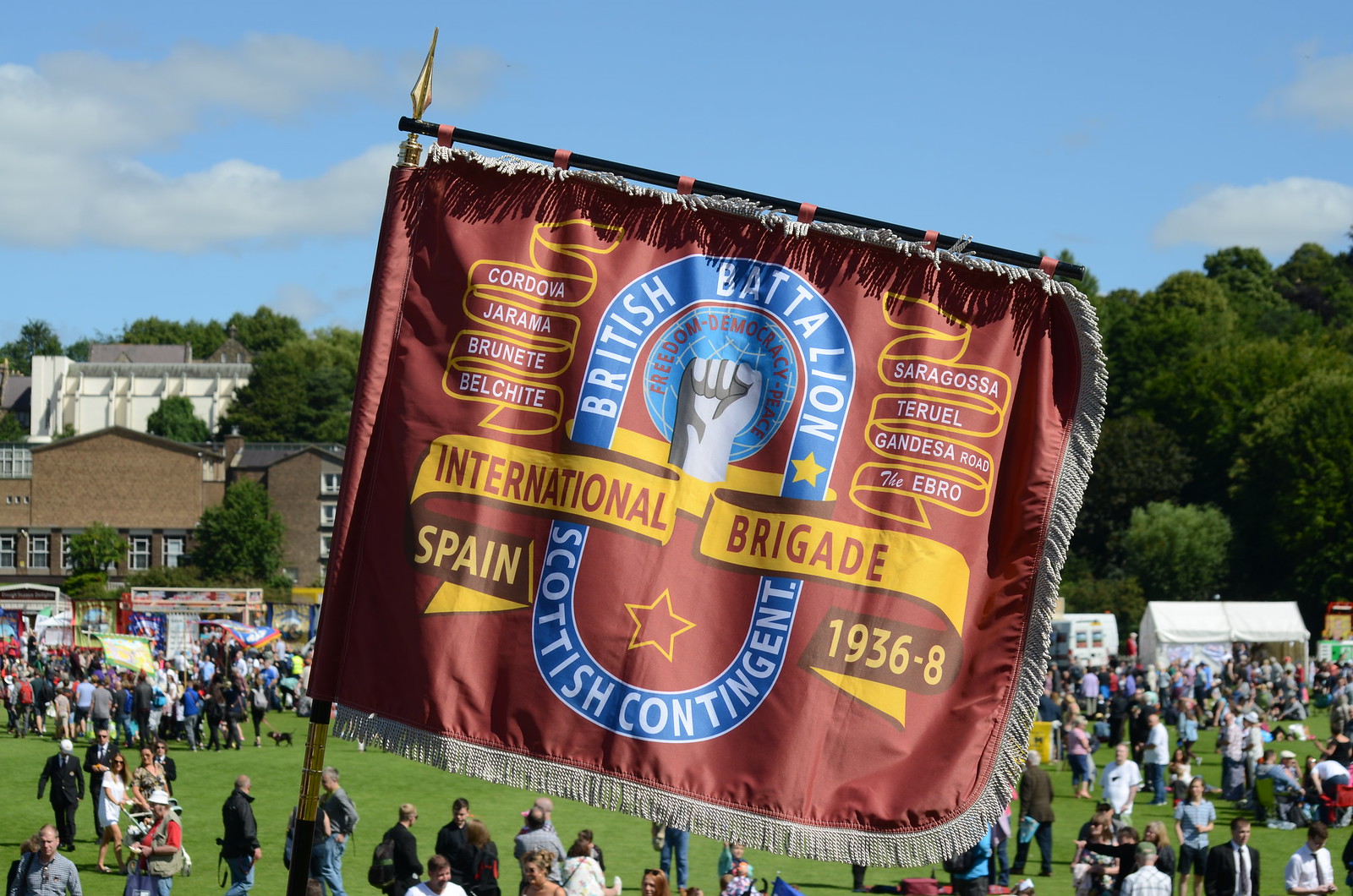The image showcases a prominent flag centered within a large, grassy field filled with over a hundred people. The flag, adorned with various colors such as brown, blue, yellow, white, gray, red, light blue, maroon, black, and green, features a hand graphic in the middle with an emblematic ribbon and text around it. The text reads "British Battalion, Scottish Contingent," encircling the hand graphic, and below it are the words "Cordova, Jarama, Brunete, Belchite, Saragossa, Teruel, Gandesa, the Ebro, Spain, 1936-8." The flag also has a yellow ribbon with the text "International Brigade, Spain, 1936-08" and a blue ring with white text specifying "British Battalion, Scottish Contingent."

On the left side of the flag, there is a ribbon graphic with the word "Spain" beneath it, while on the right, another ribbon graphic holds more text with the dates "1936-8" below. The flag is attached to a flagpole with support beams ensuring it is always flat and visible. Surrounding the flag, numerous people are seen enjoying an outdoor event, possibly on a college campus or in a large open park, with tents, food stalls, or carnival attractions scattered around. In the background, there are trees, a few buildings, and a blue sky dotted with white clouds, suggesting it's a clear, sunny day.